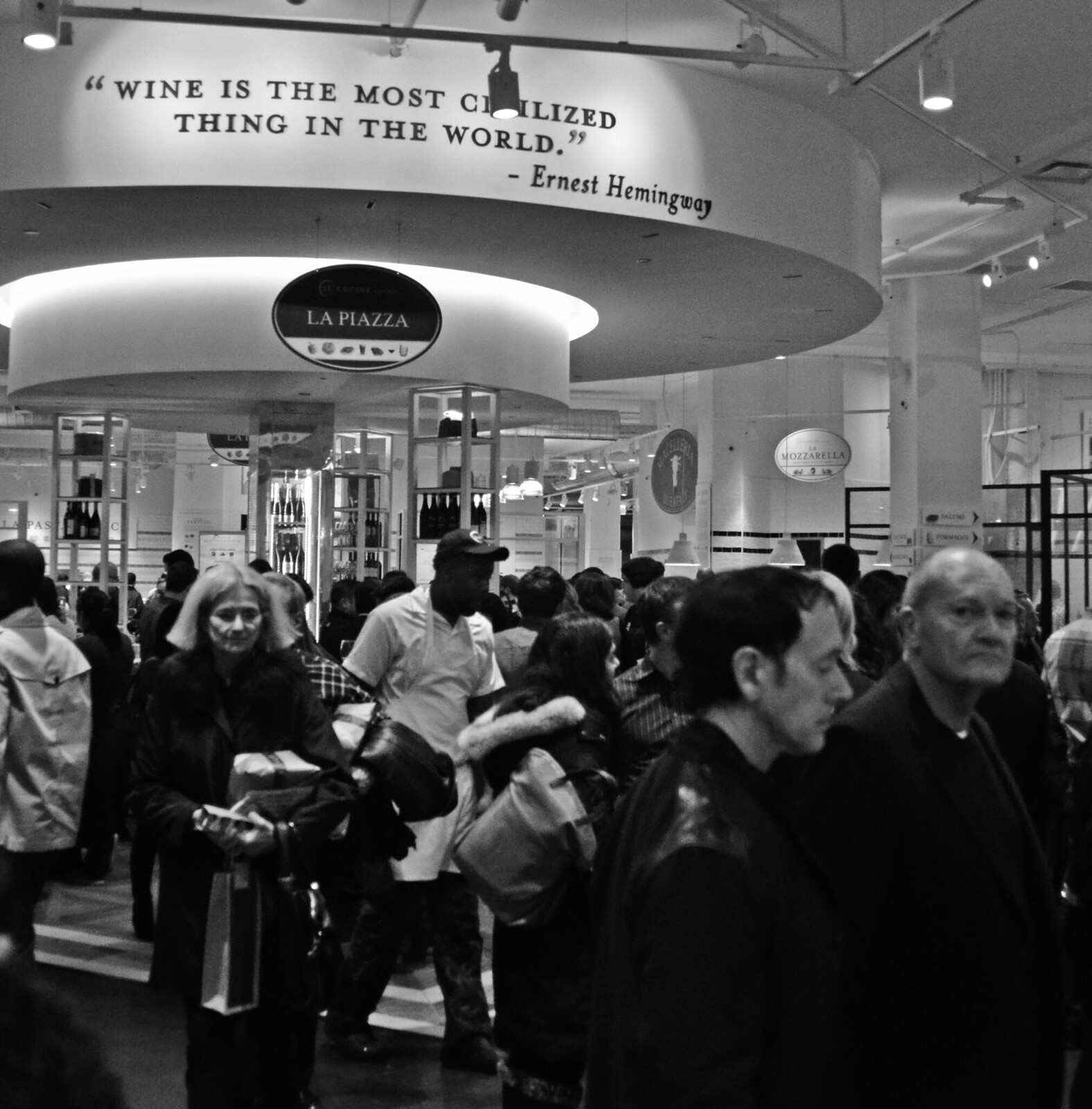This tall, rectangular black-and-white image captures a bustling indoor mall, perhaps a market or train station with shops, swarming with people. In the bottom half, the crowd is composed of diverse individuals, fully visible or from the torso up. Noteworthy figures include a black man in a hat and white shirt, a woman holding bags, and a bald man looking toward the photographer. The top of the image reveals a ceiling adorned with long metal poles lined with tiny cylindrical white lights. To the left, a circular disc displays a quote in all-capital letters: "WINE IS THE MOST CIVILIZED THING IN THE WORLD - ERNEST HEMINGWAY." Below, a smaller black oval sign reads "La Piazza," indicating a wine shop on shelving beneath it. Surrounding the shop, multiple shelves and columns exhibit various wine bottles and other items, while numerous eatery signs, including one for mozzarella, are visible along the right wall. This detailed depiction of the scene highlights the myriad of people moving about, engaged in their activities within this lively, structured setting.